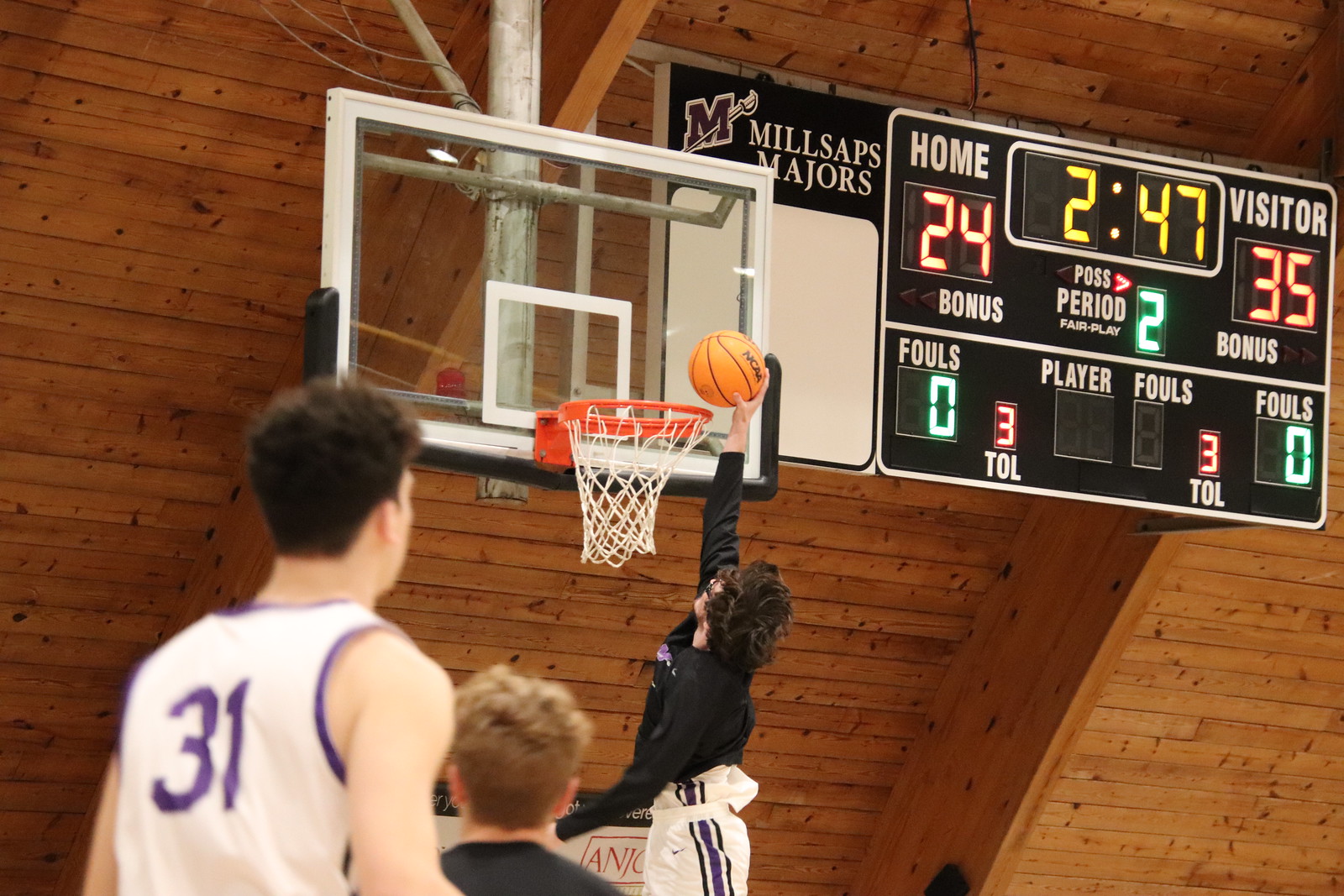This photo captures an intense moment in a basketball game, featuring three teenage boys on the court. The centerpiece of the action is a white male with long bushy hair and glasses, leaping up to score with an orange basketball. He is dressed in a long-sleeve black t-shirt and white shorts with gray and blue stripes. Next to him, a player wearing number 31 in a sleeveless white tank top looks on. The gymnasium, with its distinct sloped wooden ceiling, provides a dramatic backdrop. Prominently visible to the right of the orange-and-white basketball hoop is a scoreboard displaying "Millsap Majors," with the home team leading 24 to the visitors' 35, and 2 minutes and 47 seconds left in the second period. The scoreboard also notes that there are no current fouls and both teams have three total fouls.